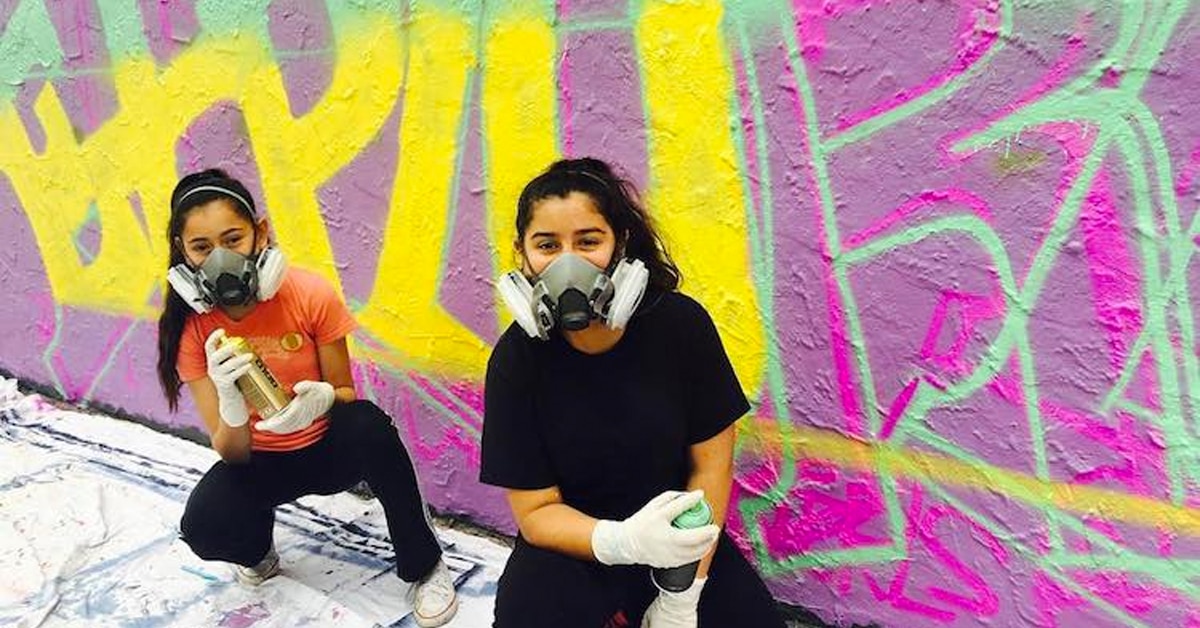In this detailed, daylight photo set outdoors, two young women with dark hair, possibly sisters, are seen engaged in a graffiti art project. They are squatting in front of a wall already adorned with vibrant and colorful spray-painted graffiti, including yellow letters on a purple background, green letters, and splashes of pink, aquamarine, and other hues. The wall appears to be wooden, and a drop cloth is laid out on the ground beneath them to catch excess paint. Both women are dressed in protective gear, wearing white gloves and substantial breathing masks with large filters on either side. One of the women, clothed entirely in black, complements her ensemble with white tennis shoes, while the other sports an orange shirt paired with black pants and white tennis shoes. Their eyes display a gleeful expression as they hold their spray cans, poised to add their finishing touches to the wall. The scene suggests they are participating in an art class or a community project.